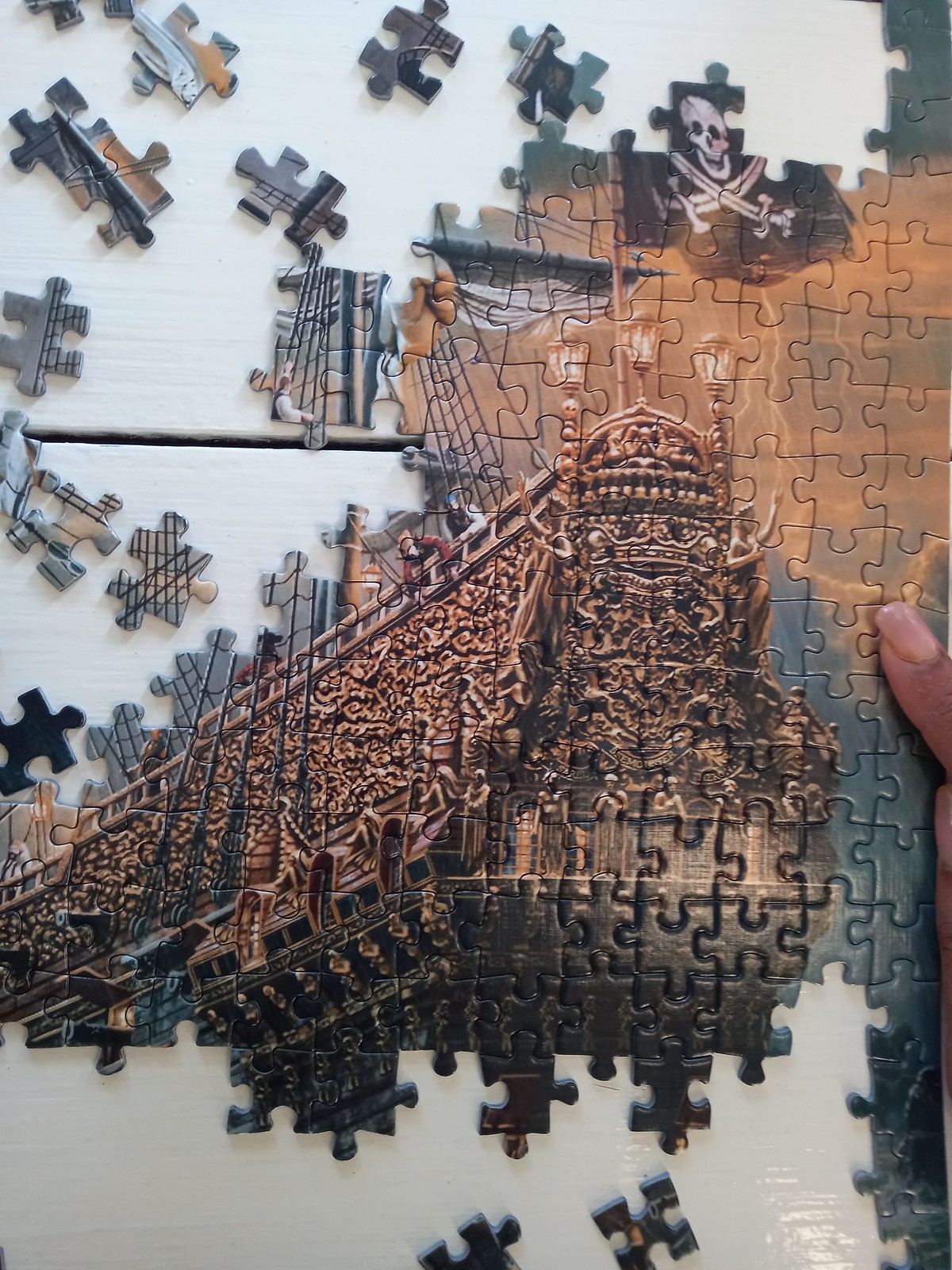This overhead photograph features a highly detailed jigsaw puzzle in the process of being completed on a white table. The central subject of the puzzle is an ornate pirate ship, depicted in a painting style with intricately carved details and a striking black Jolly Roger flag featuring a skull and cross swords on the mast. Amidst the partially assembled brown and black pieces, a human thumb is visible to the middle right of the photo, emphasizing the meticulous nature of the assembly. Scattered, face-up spare pieces add to the sense that this image was carefully arranged, possibly for social media. Although the puzzle isn't finished, the assembled sections beautifully illustrate the pirate ship amid dark blue waters, suggesting an adventurous scene, perhaps even a battle, based on the pirates and activity depicted aboard the ship. The clean and organized presentation of the puzzle elements on the pristine white surface highlights the dedication put into this captivating and visually rich pastime.